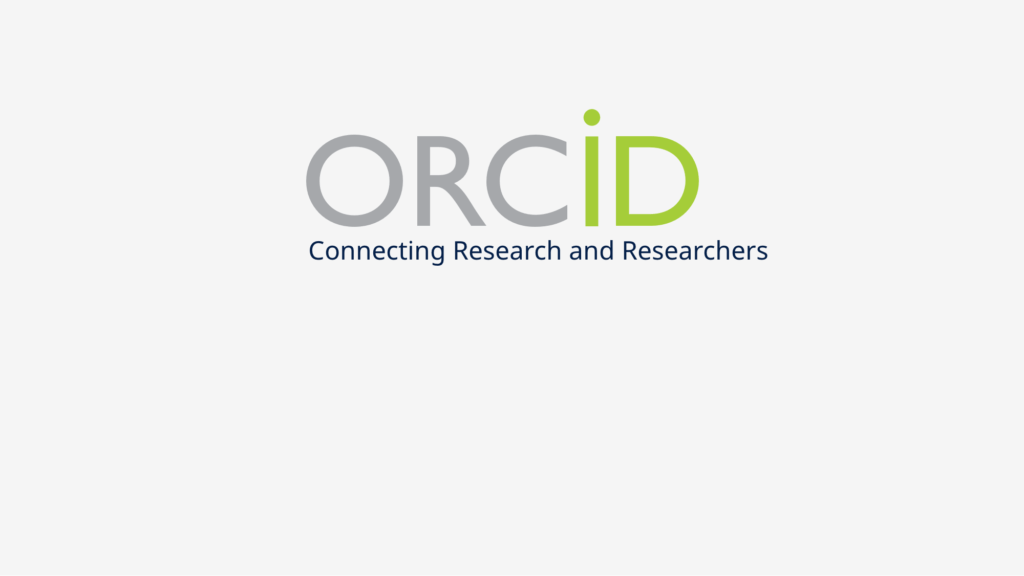This screenshot from a website features a digital advertisement set against a uniform, slightly off-white background. Dominating the upper center of the image, the word "orchid" is displayed in large, clear font. The letters "O," "R," and "C" are rendered in a light silvery gray, while the letters "I" and "D" are in a light lime green, adding a subtle contrast. Directly beneath this word, the tagline "Connecting Research and Researchers" appears in a royal blue font. The tagline is almost centered but leans slightly to the right, making the composition appear somewhat skewed and unfinished. The "C" in the tagline aligns almost directly under the "O" of "orchid," creating an imbalance that detracts from the overall visual appeal. This could potentially be a mock-up for an advertisement or a nascent design element for a website, suggesting it might still be a work in progress. Overall, the image is sparse, with only the text elements visible against the plain background.